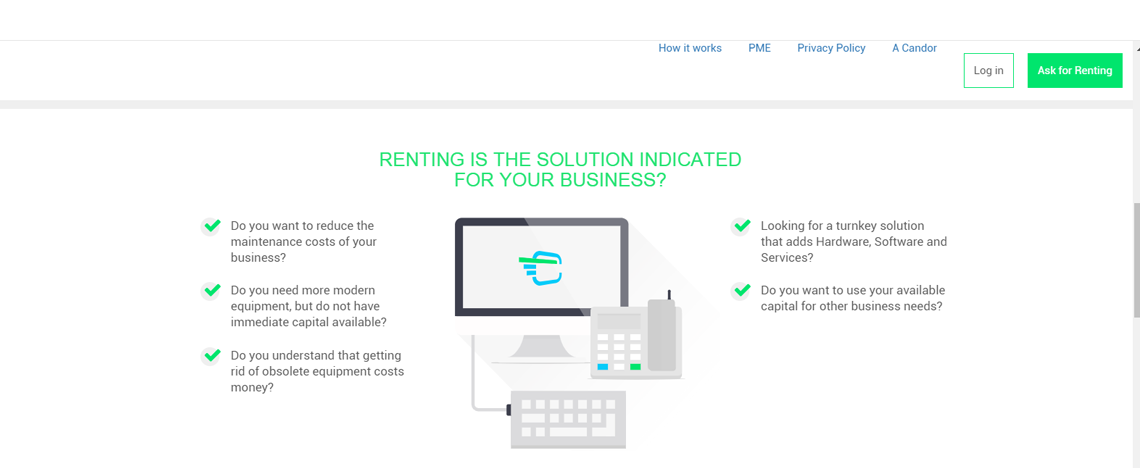The image portrays a clean, modern business website with a predominantly white background, making up about 80% of the screen, contrasted by bright, vivid colors. At the top of the page, aligned to the right in a bold yet bright blue color, are four clickable options: "How it Works," "PME," "Privacy Policy," and "About Candor." Just below these options, in the top right corner, are two buttons: a green-outlined white box labeled "Log In" and a fully green button with white text that reads "Ask for Renting."

Central to the webpage, a prominent bright green headline asks, "Is Renting the Solution Indicated for Your Business?" Below this headline, an image depicts a tablet, a phone, and a keyboard. To the left of this image, three green check marks precede concise paragraphs that address common business concerns:
1. "Do you want to reduce the maintenance costs of your business?"
2. "Do you need more modern equipment but do not have the immediate capital available?"
3. "Do you understand that getting rid of obsolete equipment costs money?"

To the right of the image, two additional green check marks introduce statements aimed at further inquiries:
1. "Looking for a turnkey solution that adds hardware, software, and services?"
2. "Do you want to use your available capital for other business needs?"

The page is laid out in a horizontal, landscape format with a strikingly modern aesthetic, defined by its minimalist design and strategic use of vibrant colors to highlight key elements.